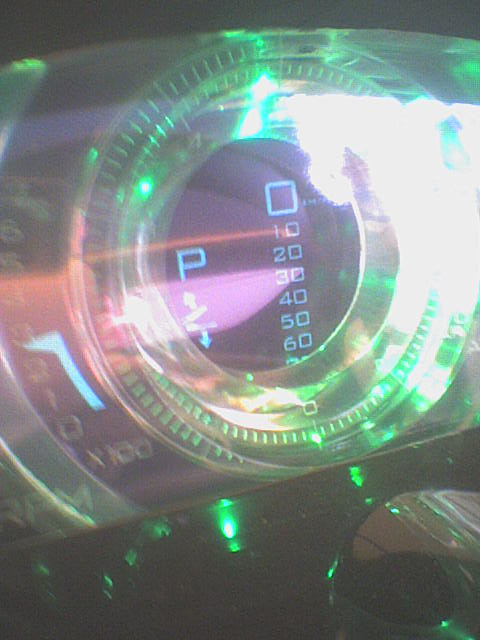A close-up, vertically-oriented photograph captures the intricacies of a car's dashboard. The image focuses on the detailed instruments and is filled with reflections, making it somewhat difficult to discern every element clearly. In the bottom left corner, the label "RPM" is displayed prominently in capital letters, followed by a scale marked "x100," with numerical values ranging from 0 to 7. Centrally positioned in the image, a blue and pink "P" is flanked by downward and upward arrows against a black background. Adjacent to this, a sequence of numbers—0, 10, 20, 30, 40, 50, and 60—is illuminated by a circular green light. The myriad of reflections across the smooth surfaces adds a dynamic, albeit slightly confusing, layer to the composition.